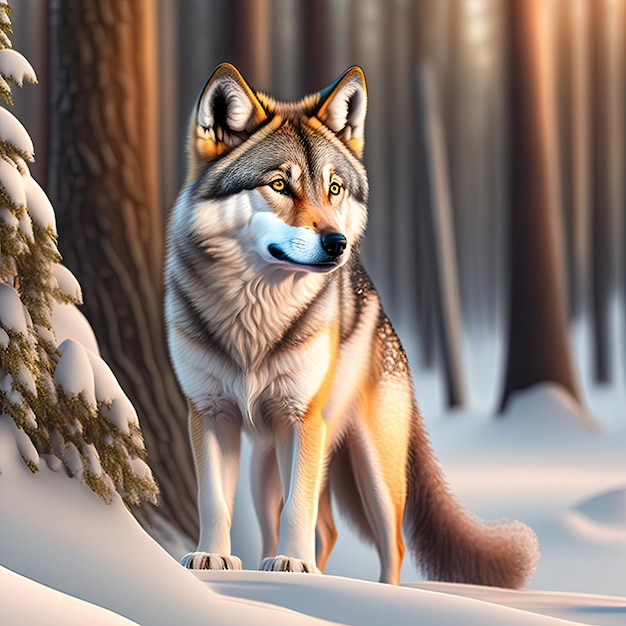This image showcases a digitally created, highly detailed and vividly colored depiction of a fox standing in a snowy winter forest. The fox, centered in the image, strikes a lifelike yet animated pose, its head turned slightly to the right, displaying its expressive yellow eyes and a striking black nose. Its fur transitions in hues from orange and tan to light brown, with white accents around its ears and mouth, and its long, fluffy tail echoing these vibrant colors.

The tranquil scene is set against a backdrop of numerous thin tree trunks, rendered in varying shades of brown, devoid of branches or leaves, which blur softly into the background to emphasize the fox in the foreground. On the left side of the image, a portion of a snow-covered pine tree adds a touch of green and a textured, wintry charm. The ground beneath the fox is a pristine blanket of undisturbed snow, enhancing the peaceful, untouched atmosphere of the forest setting.